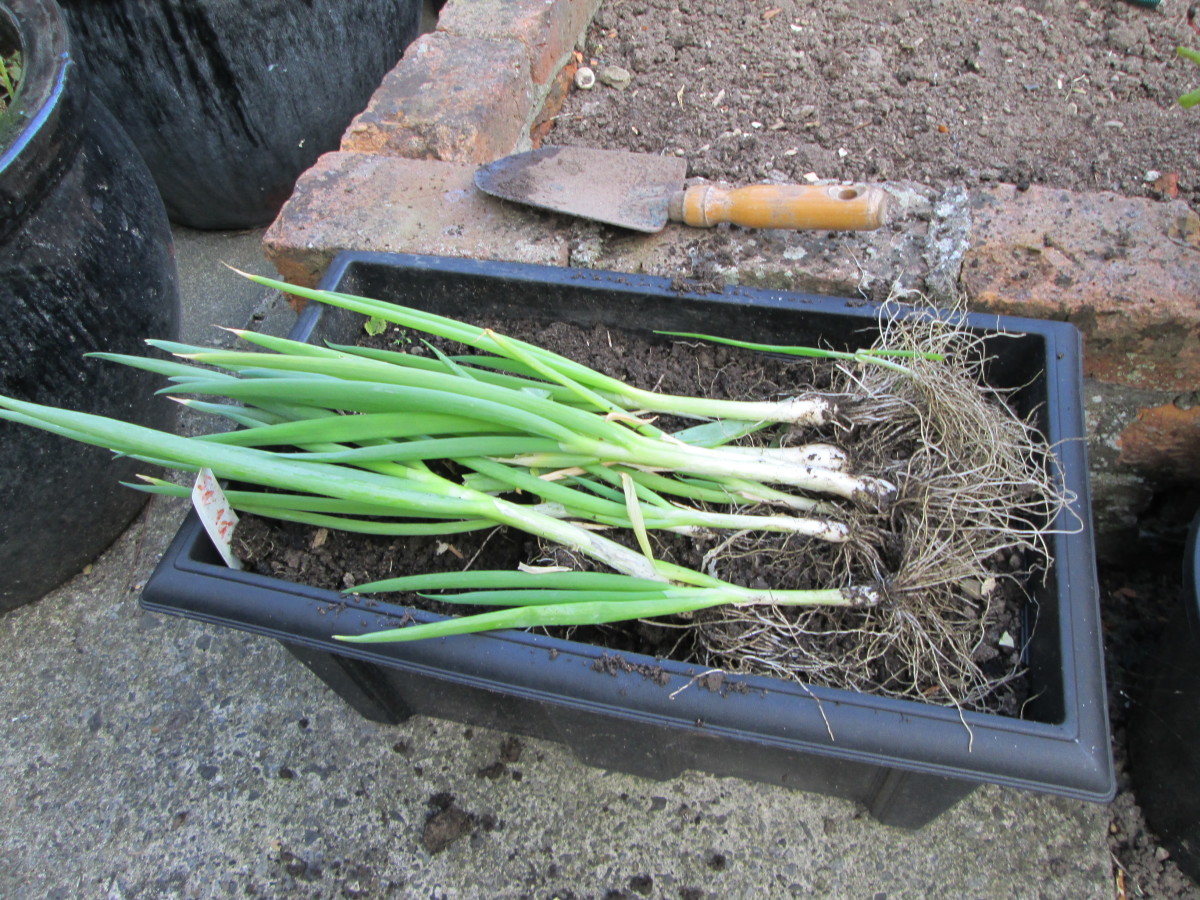This detailed landscape photograph showcases a collection of freshly harvested green onions placed on their side within a black rectangular plastic planter. The green onions, which are most likely edible, display long white stems with brown and white root tendrils on the right, and thick grass-like green leaves on the left. The plants rest on a dark bed of soil within the planter, which sits atop a flat concrete surface. A white, unmarked tag is positioned at the planter's corner. Near the top edge, a well-used wooden-handled spade lies above the onions, indicative of recent gardening activity. The surrounding environment includes additional rectangular plastic planters visible in the top left and bottom right corners, while a brick-raised garden bed filled with soil occupies the top right corner, enhancing the earthy gardening scene. The photographic style is representational realism, capturing the vibrancy and details of the freshly harvested produce and its gardening context.